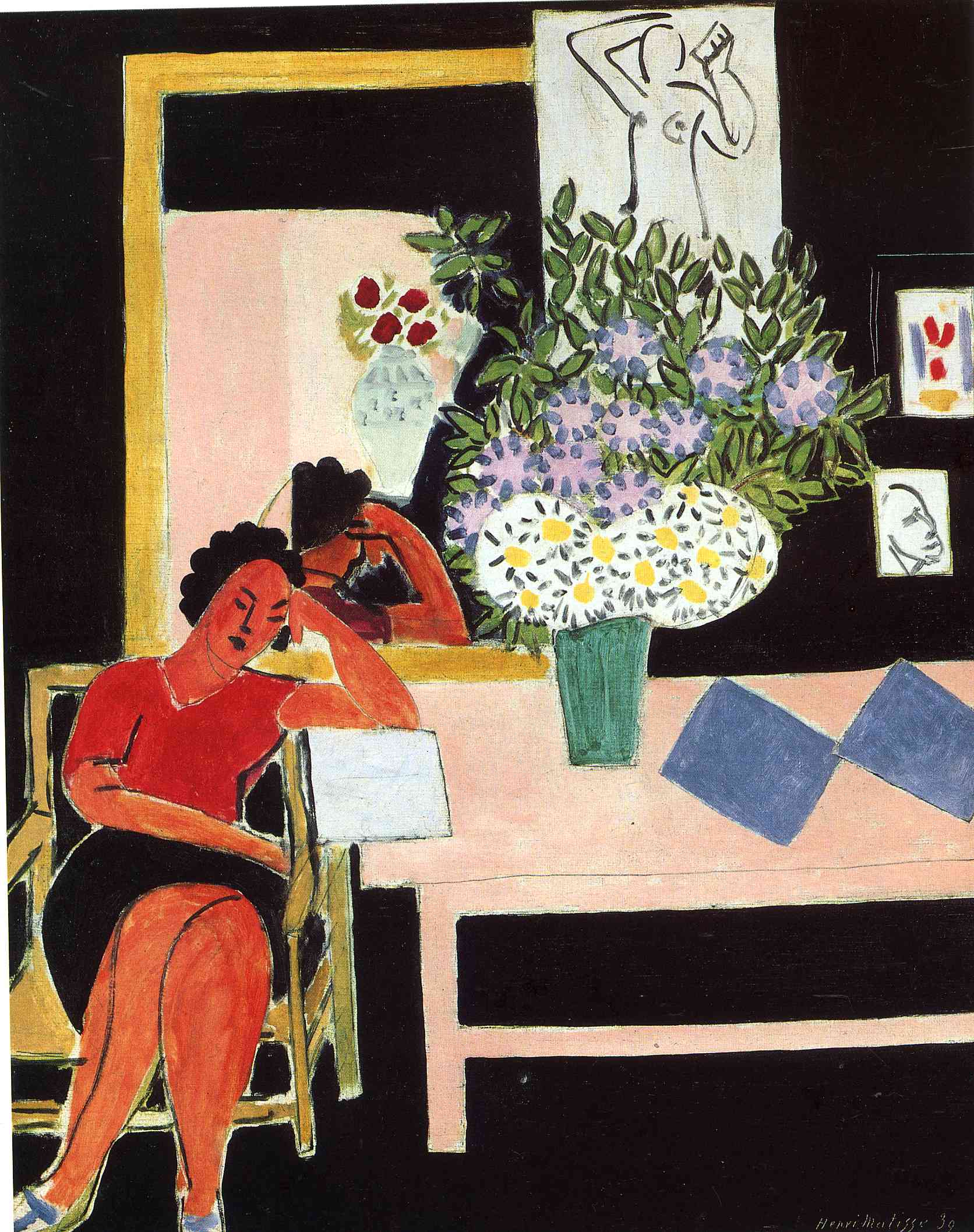An abstract art piece portrays a woman seated in the bottom left of the composition. She wears a red blouse, a black skirt, and green and blue shoes, sitting cross-legged with her right arm rested on a light pink table and her left hand supporting her head. She has black curly hair and her skin is colored in orange tones. Behind her, a mirror reflects the back of her head and arm. On the pink table is a vase containing a variety of flowers, including white daisies with yellow centers, pink and purple blossoms, and green leaves. Also on the table are two blue diamond-shaped objects, possibly napkins. The background, which is predominantly black, features several framed pictures and portraits. At the top, there is a line drawing of a person holding an object. Below it, an abstract painting consists of red, blue, and yellow brush strokes on a white background. Another line drawing of a figure's face appears further down. The overall art style employs markers, colored pencils, and other simpler drawing techniques, giving the piece a distinctive and vibrant composition.